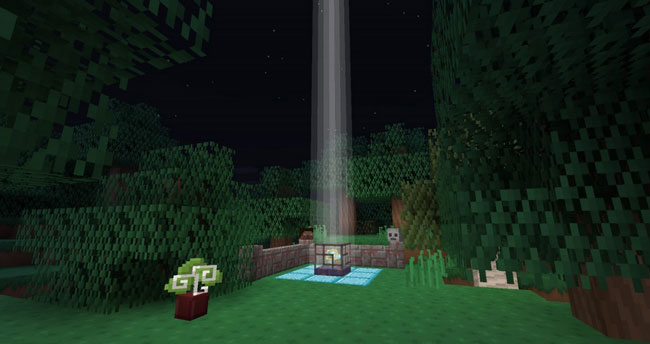This image is a nighttime screenshot from Minecraft, showcasing a distinctive in-game scene. The dark atmosphere reveals no sun, with mobs respawning more frequently and even non-hostile mobs turning hostile. The center of the image features an altar-like structure, illuminated by a bright white spotlight that pierces the night sky. Surrounding this centerpiece are columns and diamond blocks, adding to the altar’s mystique. Adjacent to it, on the left, is a peculiar object resembling a mushroom with a 'cheese sap.' The ground around is a vivid green, representing grass, and is flanked by pixelated trees and shrubs, all characteristic of Minecraft’s iconic blocky aesthetic. To the right, there’s a brown trunk, while the left side showcases a potted plant with a brown base, light green leaves, and white vines. The overall scene, framed in green foliage, captures the whimsical yet structured nature of the Minecraft world.